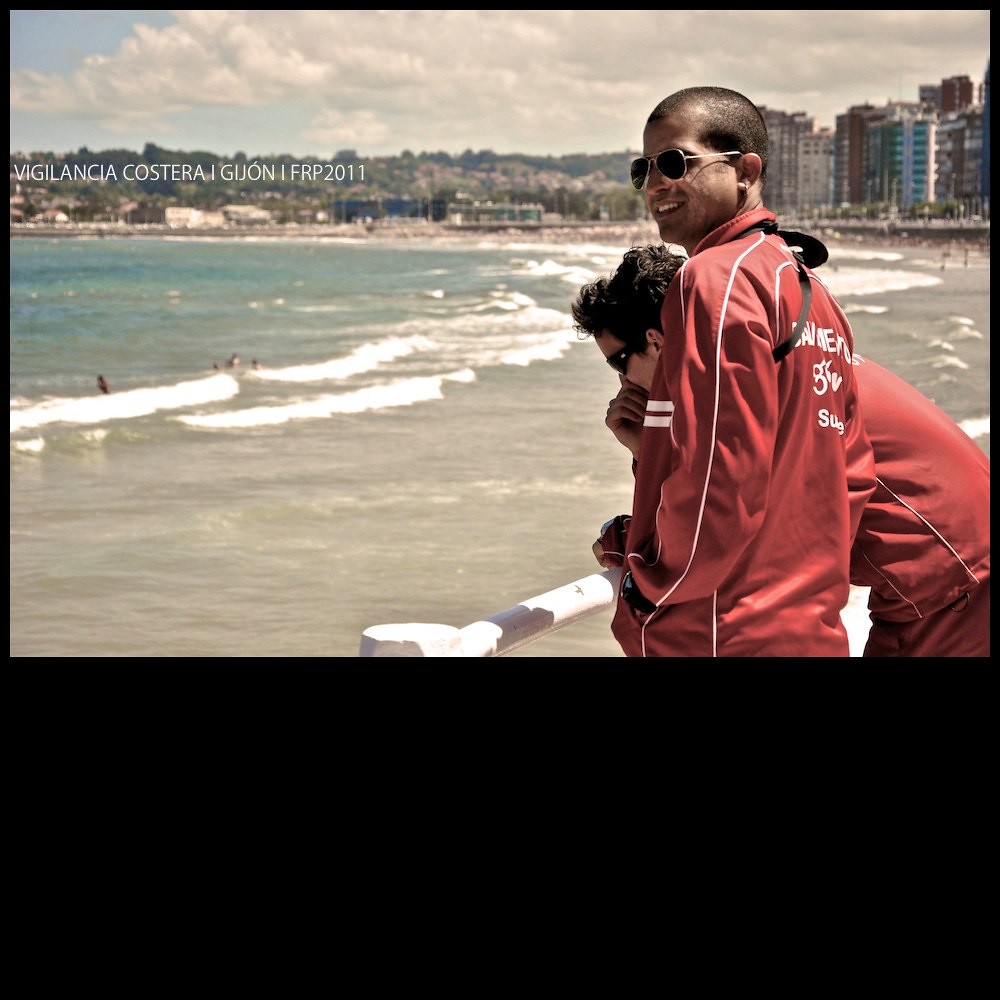This is a detailed image of two lifeguards, identified by their matching red uniforms and the white text on their backs that reads "Vigilancia Costera Guijan FRP 2011," overlooking a bustling beach scene. Both lifeguards are dressed in red track jackets and pants, featuring white piping on the sleeves, edges, and backs, as well as two white stripes across their chests. They also sport their collars turned up. The lifeguard in the foreground, with closely shaved brown hair, is wearing silver metal sunglasses with black frames and is looking off to his left with a smile on his face. The other lifeguard, with thick brown hair, is leaning on a white railing, hand cupped over his nose and mouth, wearing black sunglasses. 

The scene is set against a backdrop of a busy beach where people can be seen enjoying the sand and the ocean waves. On the left side of the image, there's a clearer view of the beach with sand and the ocean. You can also see trees and a hill in the distant background. To the right, tall concrete buildings are visible, suggesting a densely populated area right behind the beach. The image, which has an outline in black and a large black strip across the bottom, captures a moment of vigilance and relaxation as the lifeguards oversee the safety of beachgoers from an elevated position behind a white, cylindrical pole fence.